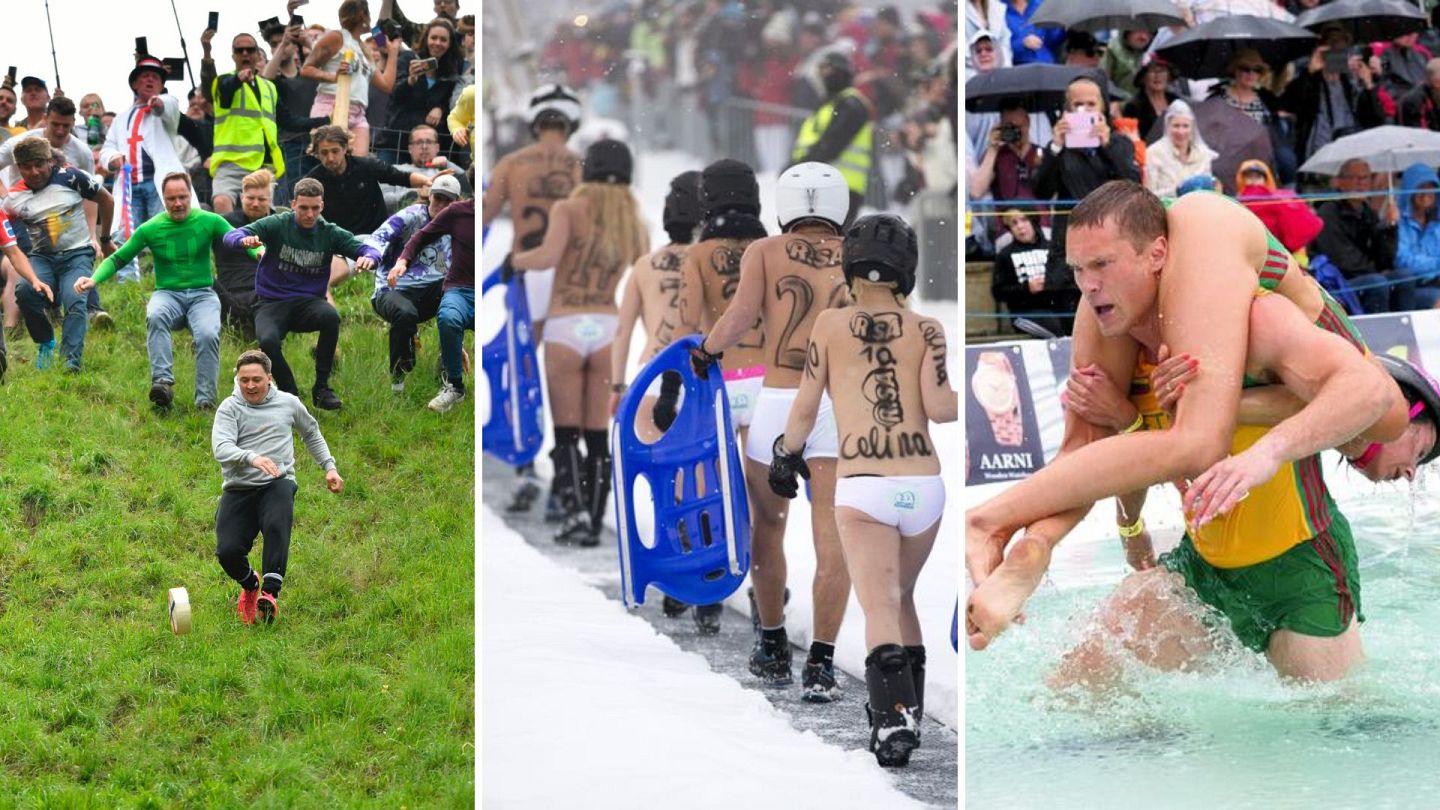The image comprises three photographs, each depicting a unique event. On the left, there is a scene of a grassy, sloping hill crowded with people, some running downhill towards what appears to be a rolling object resembling a dial or chip. The participants vary in age, with some possibly in their 30s or 40s, and the atmosphere is energetic as others at the top cheer them on. The middle photograph shows a group walking on a narrow, dark green path bordered by snow, all dressed only in underwear with tattoos and numbers visible on their backs; they might be carrying a bobsled and are braving the cold in these skimpy outfits, suggesting camaraderie and endurance. The rightmost photo features a water sport where a man stands knee-deep in water, balancing another person on his shoulders. This secondary person is draped with their legs around the first individual's head, and onlookers stand behind them, observing the activity. The shared elements across the images emphasize physical challenge and a communal spirit in diverse, adventurous settings.